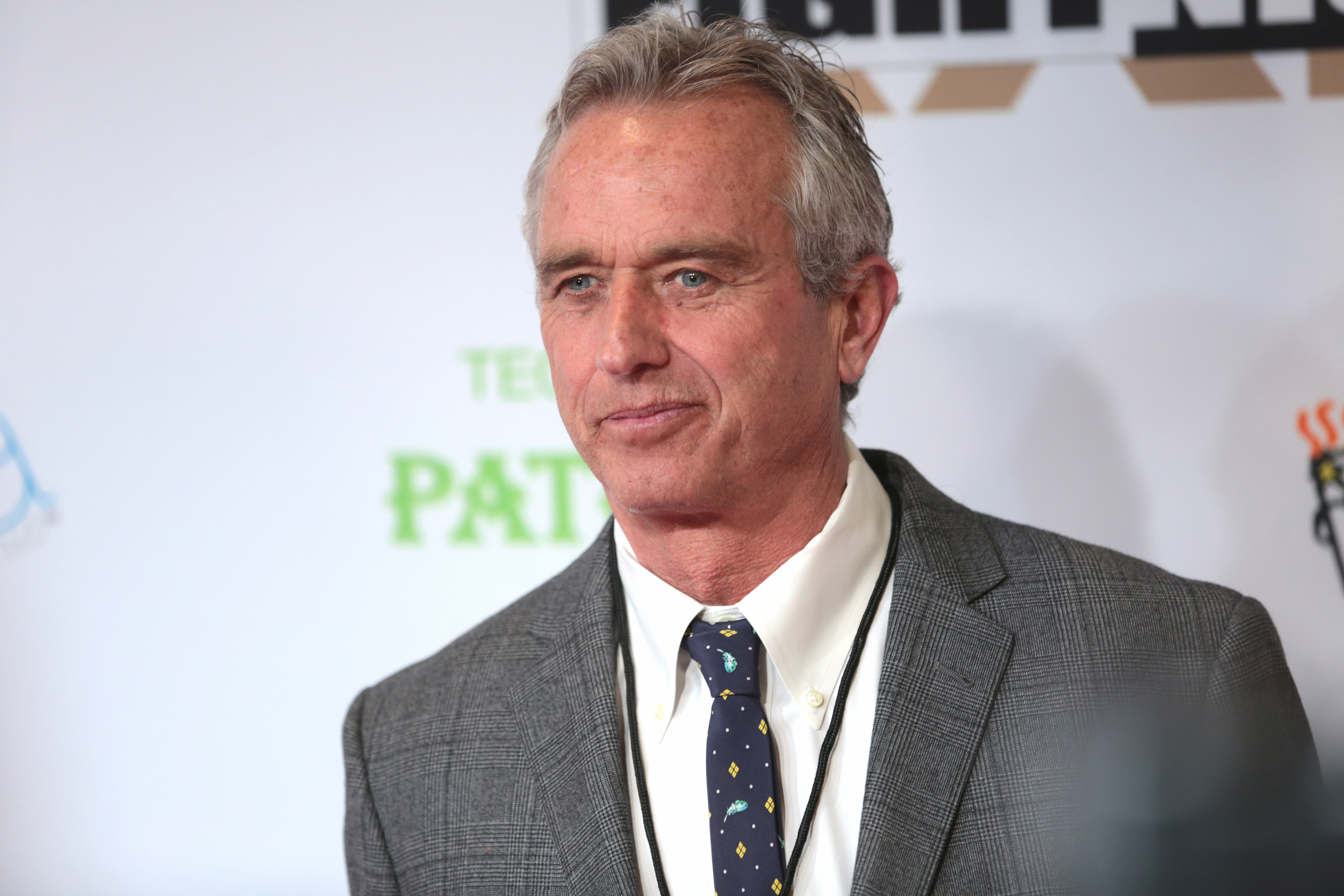A detailed photograph showcasing Robert F. Kennedy, a 2024 U.S. presidential candidate and member of the famous Kennedy family, captured against a white backdrop with the word "TELPAT" in bold capital letters in the background. Kennedy is dressed in a dark gray suit jacket paired with a crisp white collared shirt. Adding a touch of whimsy to his formal attire, he sports a navy blue tie adorned with yellow sparkles and magical shapes, reminiscent of comet-like patterns. His attire is completed with a neck strap, possibly holding an ID card, indicating his attendance at a special or celebrity event. Kennedy, a Caucasian man with light skin, is depicted with a very slight smile on his face, casting a subtle shadow on the wall behind him. The photograph captures his poised and approachable demeanor.